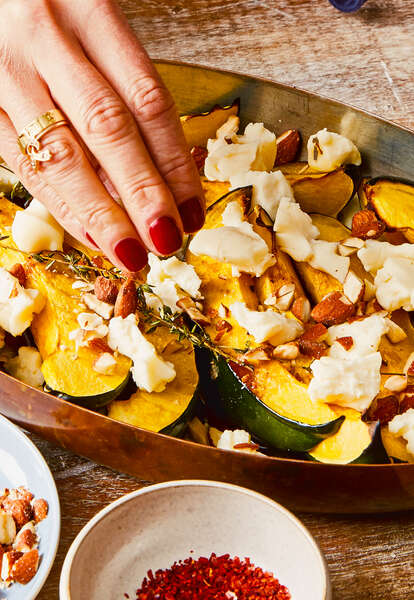In the photograph taken indoors, a detailed culinary scene unfolds. At the center, an elongated wooden dish holds a medley of roast acorns, strewn with slices of green apples, sprigs of parsley, and globs of cheese, possibly brie. From the top left corner, a hand, adorned with red nail polish and a gold wedding band, reaches down to grasp the food. This hand, wrinkled with age, suggests it belongs to an older woman. Below the main dish, positioned on a wooden tabletop, lies a small white bowl filled with red chili flakes. To the left of it, another bowl contains an assortment of nuts. In the top right corner of the image, a blue knob or dial, possibly part of another piece of dishware, subtly peeks into the frame. This intricate composition is characterized by an earthy, inviting ambiance.